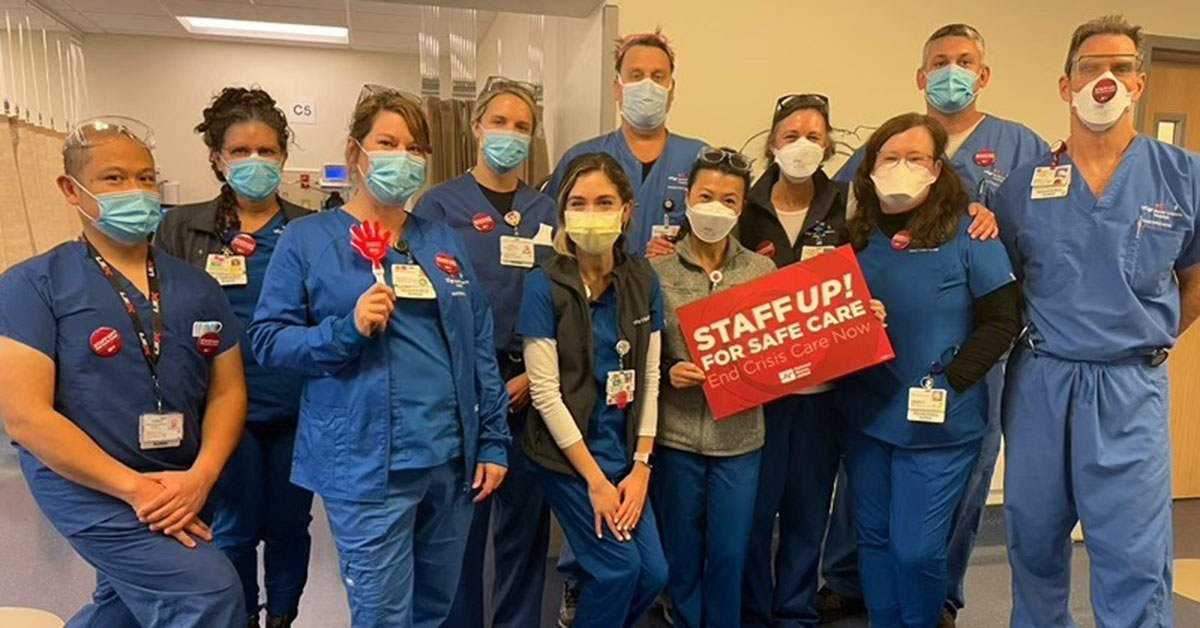In this photograph, a group of hospital staff members, comprised of nurses and doctors, stand together in what appears to be an emergency room hallway. They are dressed in various shades of blue scrubs, with most wearing blue masks, though a few have yellow or white ones. Several staff members also have glasses perched on top of their heads, and some are holding little red hand clappers. A few are wearing additional layers like gray jackets or long-sleeved shirts underneath their scrubs.

Prominently, one female staff member in a gray fleece jacket holds a red sign that reads "Staff Up for Safe Care" and "Crisis Care Now," highlighting their advocacy for workplace safety and patient protection. Additionally, many staff members display red pins on their scrubs or masks, further emphasizing their message of promoting health and safety.

Behind them, the hospital setting is indicated by the presence of medical machinery, curtains, doors, and markings on the wall, including the letter C and the number 5. The diverse team includes individuals of different ethnic backgrounds and genders, united in their dedication to healthcare. Their eyes convey a sense of resilience and commitment, likely testifying to the long hours and hard work they endure to provide essential care.